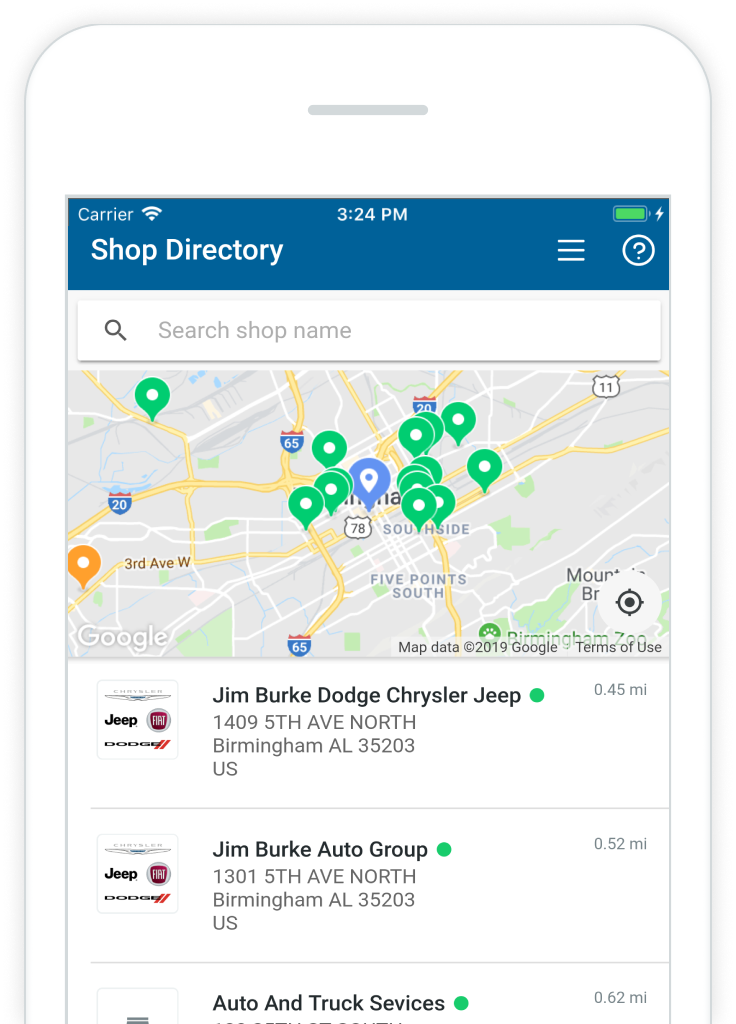The image appears to be a screenshot from a mobile application or web page used for navigation or searching for specific locations. Displayed on a smartphone with a full battery and the time reading 3:24 PM, the interface prominently features a section labeled "Shop Directory" with a small question mark icon within a circle next to it, likely for hints or help.

Below this, there's a search bar that reads "Search shop name," indicating the user can type in the names of places they wish to find. 

The central portion of the screen displays a map fragment dotted with green points or check marks, signifying various searched shops. Some annotated areas on the map include "South Side" and "Five Points South," with visible street names like "3rd Avenue W" (presumably meaning West).

Beneath the map, the app lists the search results, starting with "Jim Burke Dodge Chrysler Jeep," followed by "Jim Burke Auto Group," and then "Auto and Truck Services," though the full address of the last entry is truncated and not fully visible.